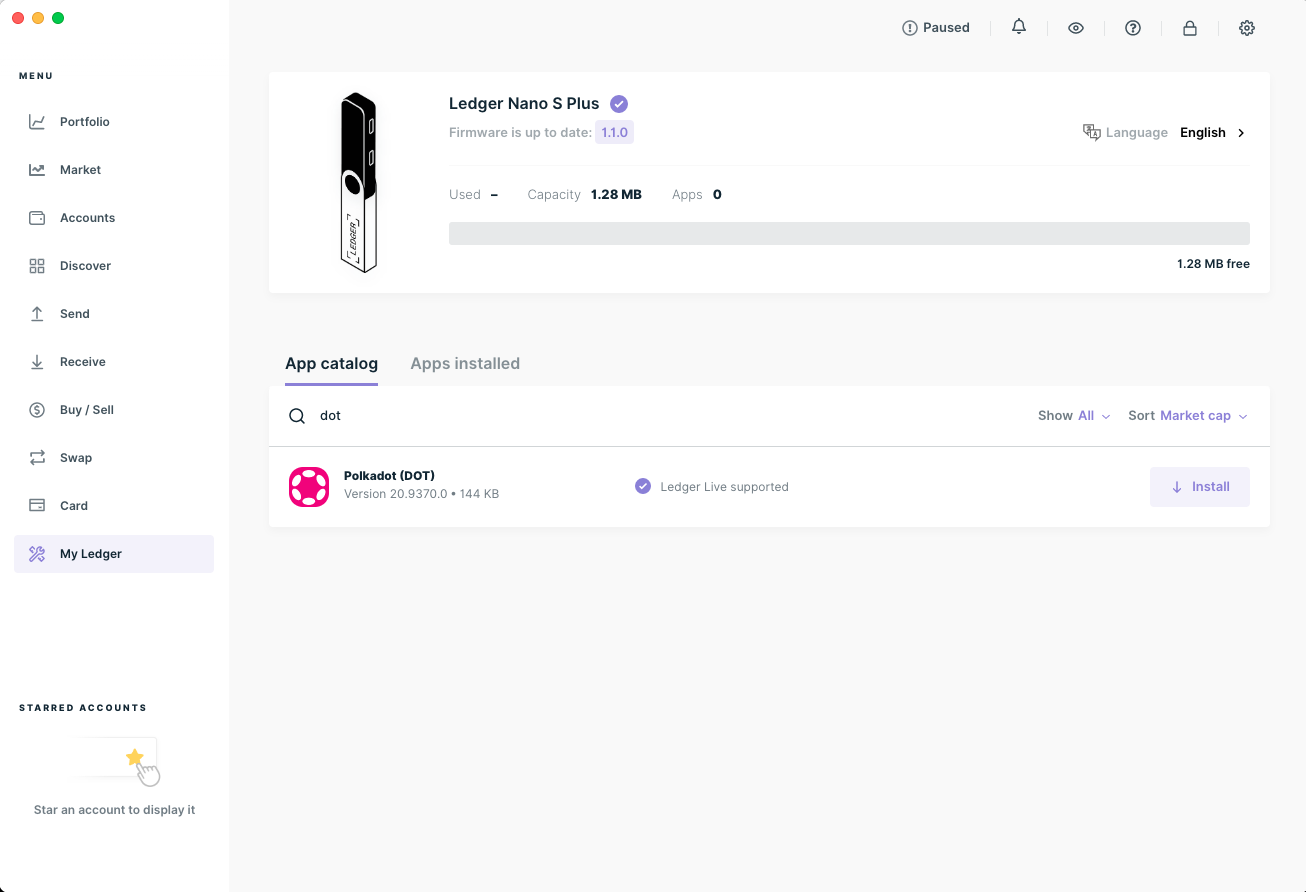Screenshot of a MacBook Air Displaying Cryptocurrency Management Interface

The image depicts a screenshot of a MacBook Air interface, identifiable by the distinctive red, yellow, and green circular buttons located in the upper left corner of the window. Below these buttons, the word "Menu" appears in black text.

Directly underneath the "Menu" text, a navigational sidebar lists several options, each accompanied by a small icon on the left:
- Portfolio
- Market
- Accounts
- Discover
- Send
- Receive
- Buy
- Sell
- Swap
- Card

A gray box with the text "My Ledger" is visible below the sidebar. 

In the central area of the interface, the words "STARRED ACCOUNTS" are written in black, all caps. Beneath this heading is a yellow star icon with a hand pointing at it, accompanied by the instruction "Star an account to display it."

To the right, another gray box is visible, containing various control and informational icons at the top:
- A "Pause" button
- A bell icon
- An eye icon
- A circle with a question mark inside
- A lock icon
- A settings icon

Beneath these icons, there is a white rectangle. On the left side of this section, a device resembling a Ledger Nano S Plus, which appears to be connected to the computer, is displayed. The device is depicted with a small purple circle containing a check mark. Below the device description, the following details are listed:
- Firmware is up to date: 1.1.0
- Used capacity: 1.28 MB, Apps: 0

To the right, additional information includes:
- Language: English
- 1.28 MB free

Further down, there are options labeled "App Catalog" and "Apps Installed," followed by a search icon and the text "DOT." To the right of this, it says "Show all" and "Sort: Market Cap."

In the lower left portion of the screenshot, a pink square icon featuring six football-shaped objects arranged in a ring can be seen. This icon is labeled "Polkadot (DOT)" with a version number "20.9370.0.144KB." A purple circle with a white check mark indicates that it is "Ledger Live Supported." To the right of this section, a small gray box with the word "Install" and a downward-pointing arrow in purple is present.

Overall, the detailed interface suggests a comprehensive cryptocurrency management tool, likely used for managing multiple accounts and keeping track of various digital assets.